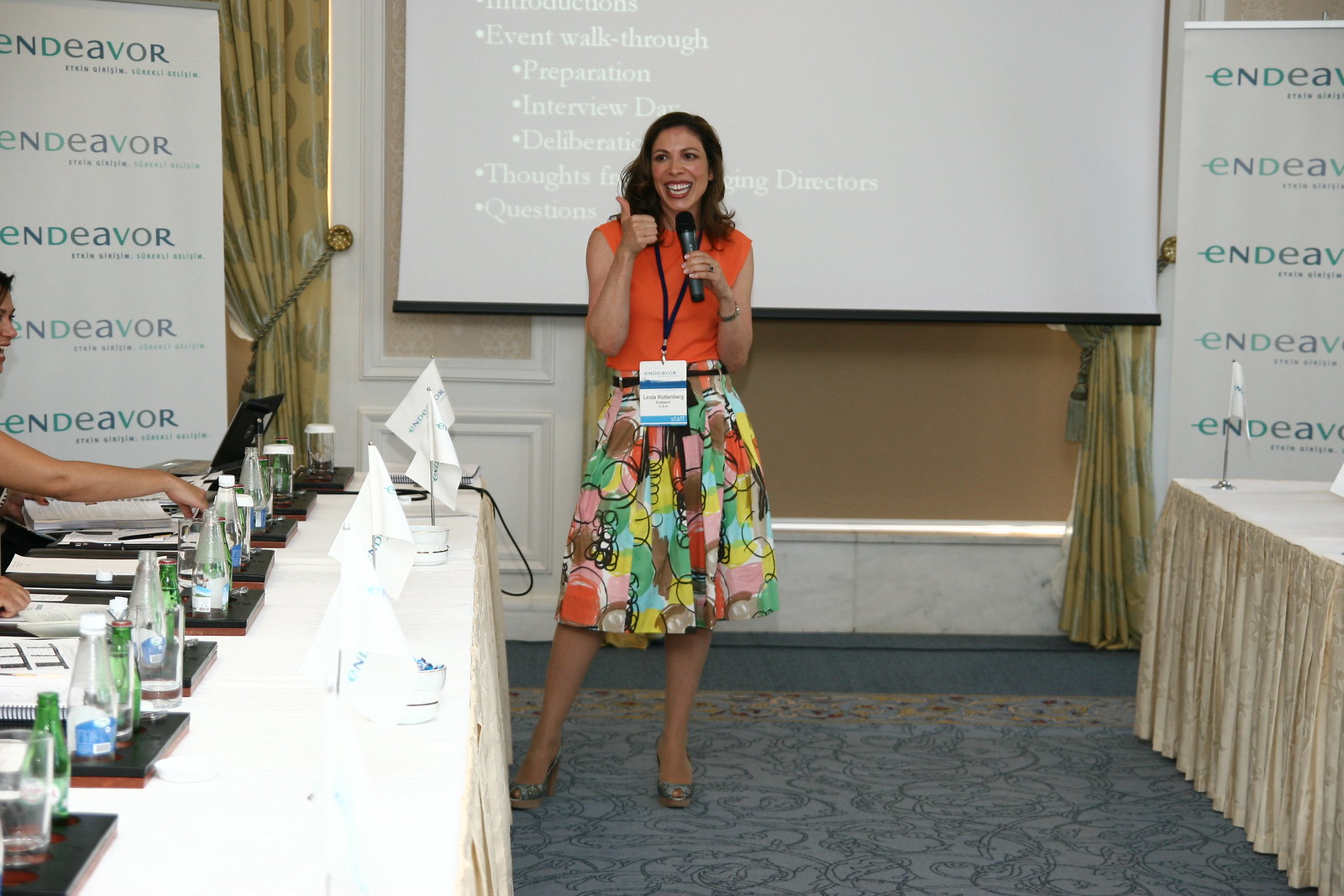The image depicts a woman with tan skin and shoulder-length dark hair, who stands confidently in what appears to be a brightly lit conference room. She is giving a presentation and holds a microphone in her left hand while giving a thumbs up with her right. Her attire consists of an orange sleeveless shirt paired with a knee-length, multi-colored skirt featuring abstract floral patterns in pinks, oranges, blues, and yellows. Around her neck hangs a lanyard with a white card. She is smiling broadly, possibly laughing, and facing slightly to the right. She is positioned in front of a projector screen that appears somewhat faded due to the room's brightness. The screen displays text reading "Event Walkthrough Preparation, Interview Day, Deliberation," with the last two bullet points partially obscured by her figure. The backdrop reveals beige, creamy-colored walls and a grey-blue carpeted floor. On her left, a long table draped in a white cloth is set with bottles of water, notebooks, and glasses. An individual is partially visible at this table, with the event branding of "Endeavor" noticeable on banners and small white flags around the room. To her right, another table is visible but partly cut off, similar in setup with water bottles and glasses. The setting and scene suggest an organized, professional environment aimed at preparation and deliberation activities.